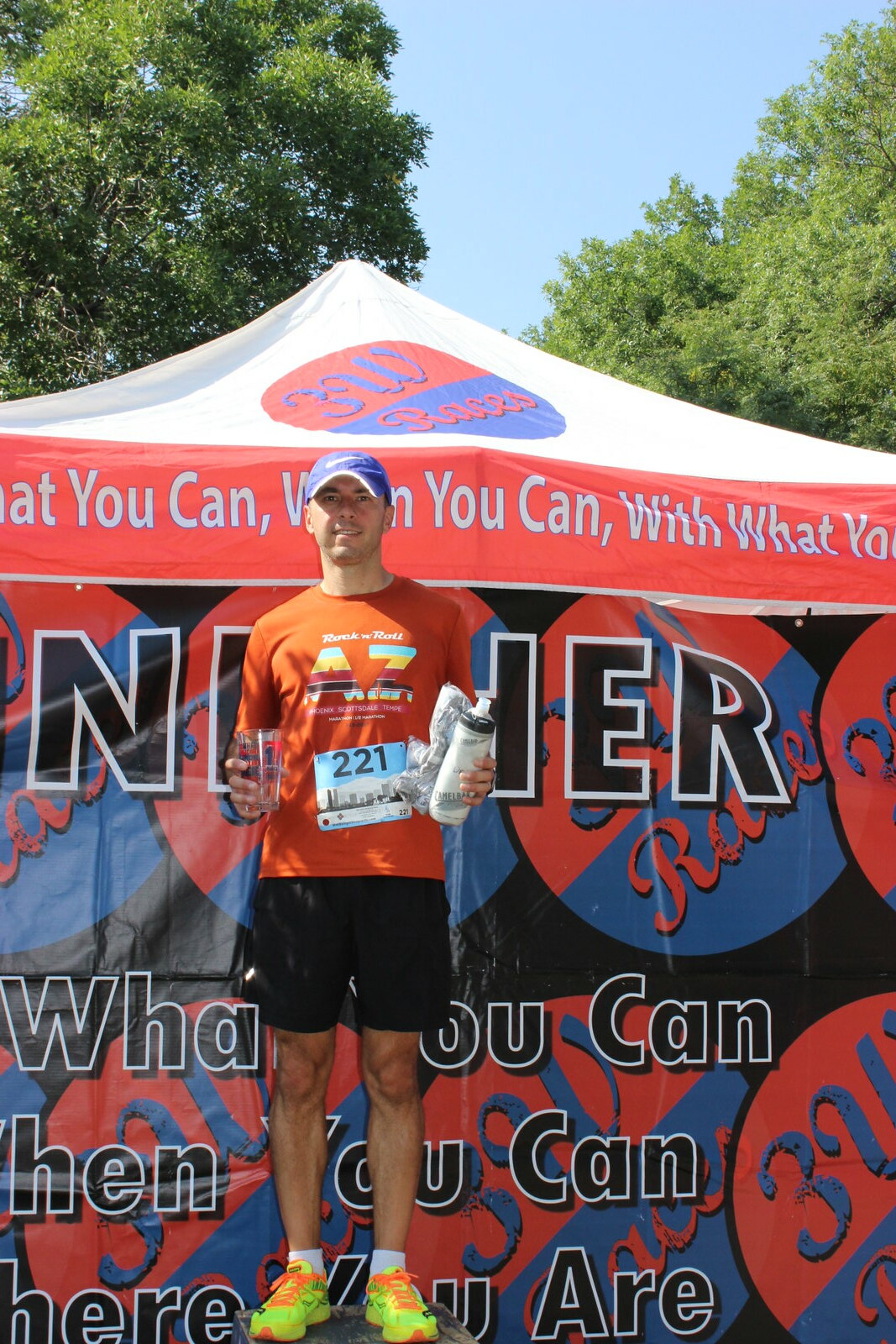A man stands proudly on a podium, likely celebrating his achievement in a competitive event such as a triathlon or a 5K run. He is dressed in black shorts, an orange shirt featuring multicolored stripes and the number 221, and wears bright yellow shoes with orange laces paired with white socks. Completing his outfit, he sports a purple cap. In his right hand, he holds a glass that appears to contain water, while in his left, he carries a water bottle and a plastic bag. Behind him is a company-sponsored backdrop, partially obscured by his presence, displaying motivational text such as "you can" and "do all you can." The man’s pose and attire suggest a moment of triumph and celebration.